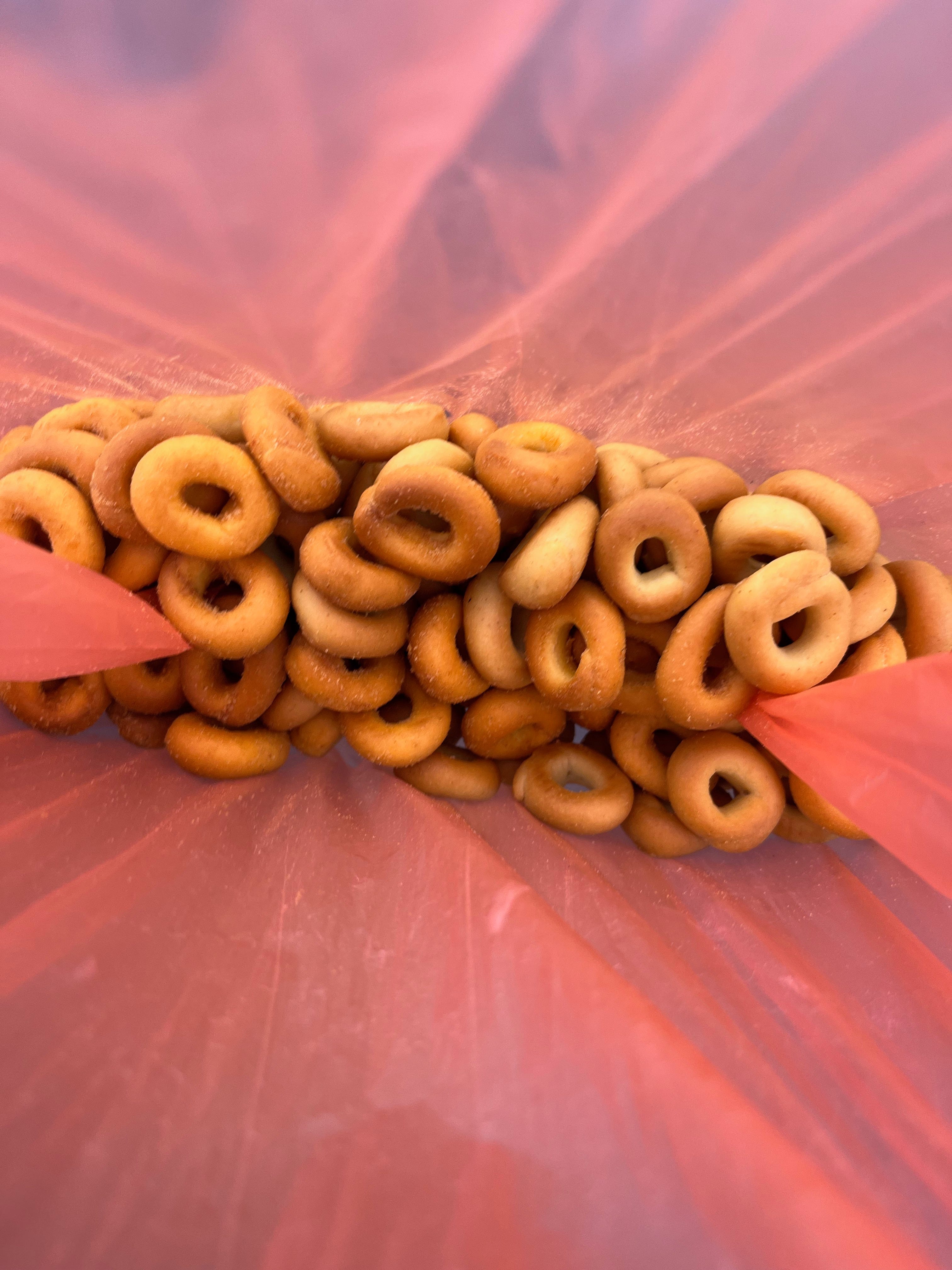The image features a close-up view inside a pinkish-red tinted plastic bag, pinched inward at the sides, revealing a collection of yellowish-brown bagels that span the bottom area of the bag. The bagels, stacked and clumped together in the center, show a toasted, brownish top with lighter beige centers, possibly sprinkled with tiny white granules. The plastic bag appears semi-transparent, offering limited visibility outside while enclosing the bagels effectively. The background outside the central cluster of bagels displays some hints of blue at the top, adding contrast to the scene dominated by the pinkish-red hue of the bag and the warm tones of the bagels.